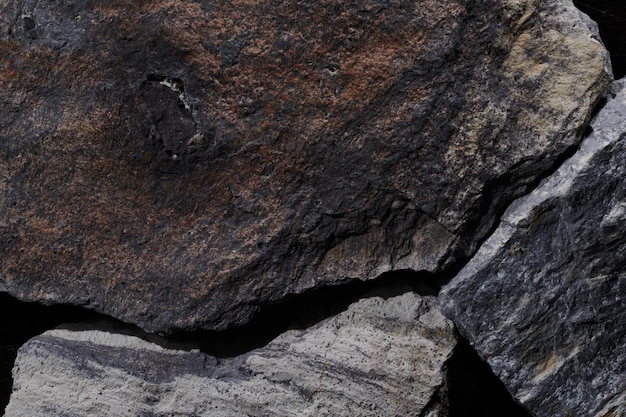The image showcases an outdoor scene featuring three large, rough-textured rocks with sharp surfaces, appearing heavy and partially broken off from a larger formation. The top rock, resting on the one below it, is predominantly gray with brown rust, black, soft tan hues, and visible cracks, with a black area behind one of the crevices. The bottom-left rock exhibits a light gray color with darker gray accents, while the rock on the right is characterized by its square edge, dark gray coloration, and a top surface that transitions to a lighter gray. The blackish-gray side of the rightmost rock faces the camera, contributing to a triangular black shading at the base. The entire composition is illuminated by outdoor lighting, although the sky is not visible.